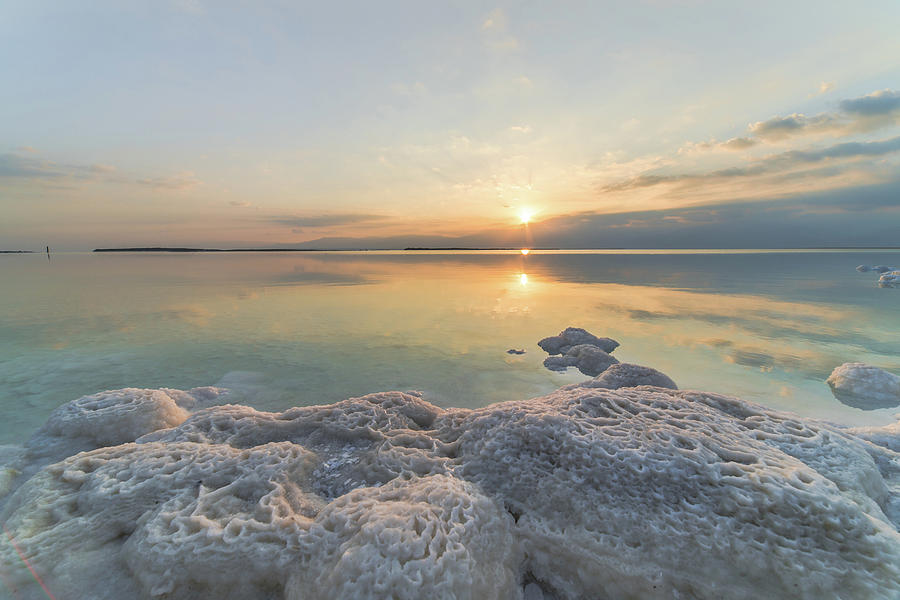The image captures a stunning sunset over a calm ocean, with a vast blue sky dotted with white and blue clouds reflecting on the water's surface. The vibrant orange sun, positioned centrally near the horizon, is just about to meet the water level, casting a warm glow across the scene. In the foreground, the photographer stands on distinctive white rocks resembling sponges or perhaps salt deposits, characterized by their lumpy texture and indentations. Beyond the tranquil waters, a series of low-lying black islands provide a striking contrast against the colorful sky. There is no text in the image, allowing the natural beauty of the sunset to speak for itself.